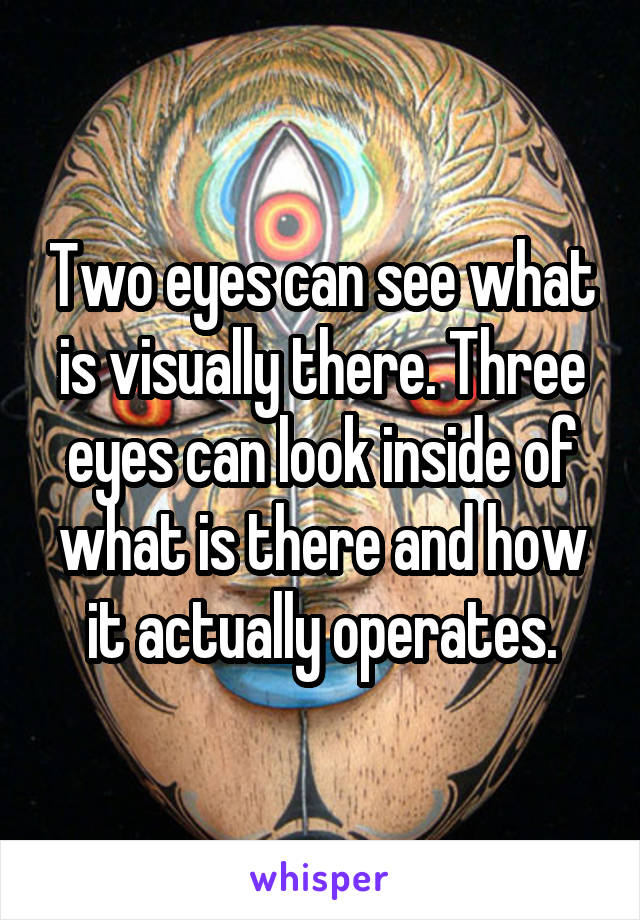The image features a highly detailed and intricate piece of art depicting a face with a fully black background. The face, rendered in flesh tones with black speckles, has three eyes: two standard eyes outlined in bright orange and red with black pupils, and a vertically oriented third eye on the forehead. This third eye has a black pupil surrounded by concentric orange and yellow rings, and is adorned with designs resembling peacock feathers in blue and green hues. The face is extensively decorated with tattoo-like patterns across the cheeks and down to the lips, which are strikingly blue. The art also includes painted eyelashes and a sharply pointed nose. Superimposed in white text bordered with black, the caption reads, "Two eyes can see what is visually there, three eyes can look inside of what is there and how it actually operates." At the very bottom, in purple text, the word "whisper" is inscribed.